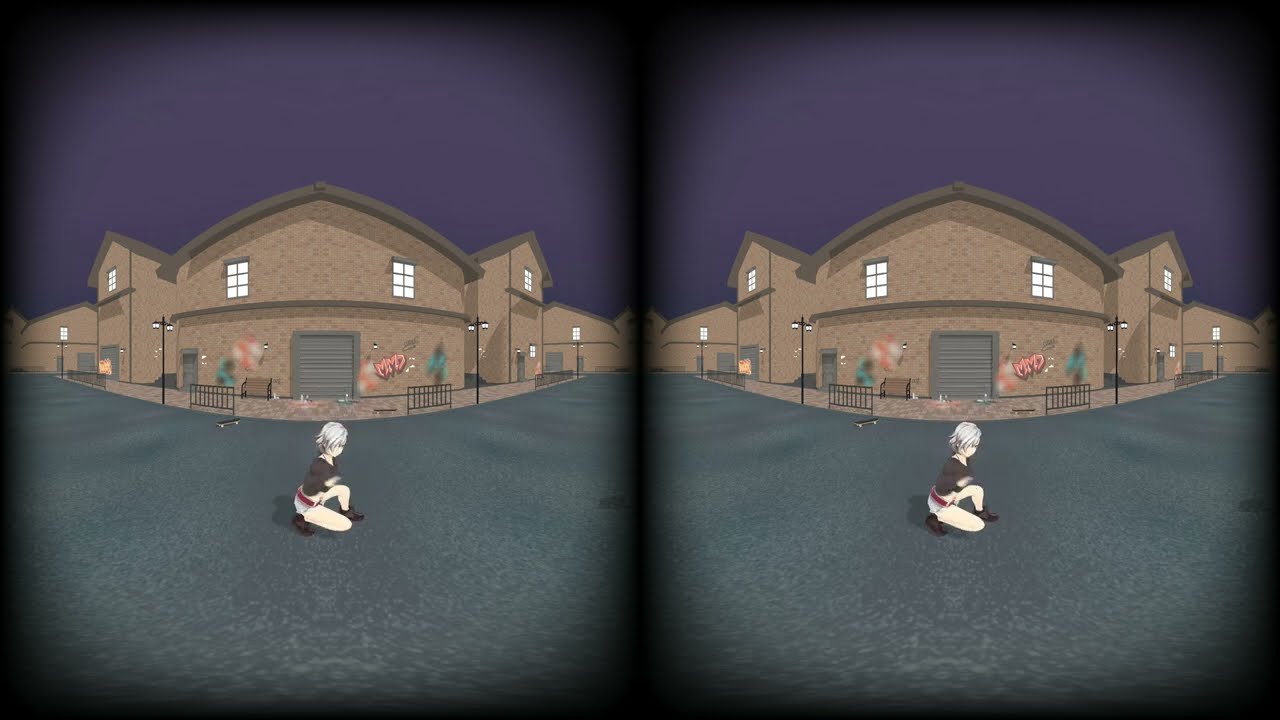The dual image showcases a detailed cartoon or artificially generated scene, presented identically on both the left and right sides. In the foreground, a cartoon woman, possibly with Asian features, is squatting on the ground; she sports gray, Lucy Liu-style hair, a black top, white shorts with a red belt, and is positioned with one knee on the pavement. Behind her, a prominent brown building dominates the background, characterized by three triangular-shaped roofs, a grand entrance, and two upper-level white windows. This structure is adorned with dark brown roof trim and has visible graffiti. Accompanying the scene are several black metal fences, street lamps, and a gray garage door, suggesting an urban setting potentially resembling a factory or commercial building.